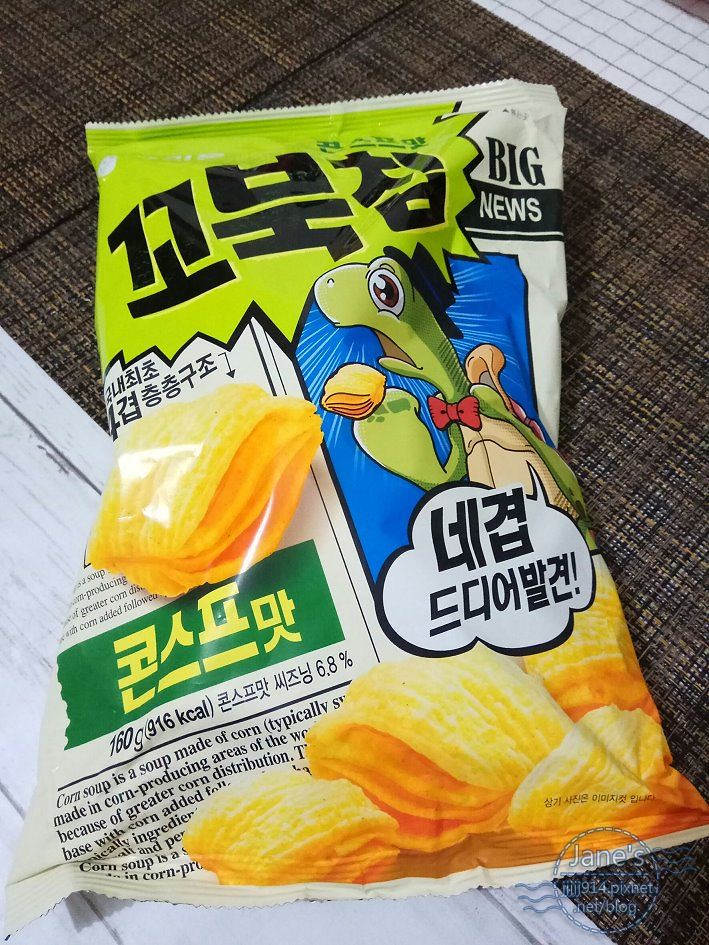The image captures a vertically-oriented photograph of a tan-colored bag of chips resting on a surface that appears to be a white wood grain tile. The bottom left corner reveals the actual tile surface, while a brown canvas-like tablecloth or runner is situated towards the top corner. The bag prominently features Asian characters within a sharp-edged speech bubble in the top left. On the upper right, the text reads "Big News," and additional text on the bottom right refers to "Corn Soup," suggesting that the chips are corn-based and possibly flavored to resemble corn soup. The lower right corner of the bag displays images of the chips, while a whimsical cartoon turtle in the middle right, adorned with a black top hat and a red bow tie, holds a stylized version of one of the chips with an open mouth. The overall setting appears to be indoors, with the image emphasizing the quirky, detailed packaging and the unique snack it contains.